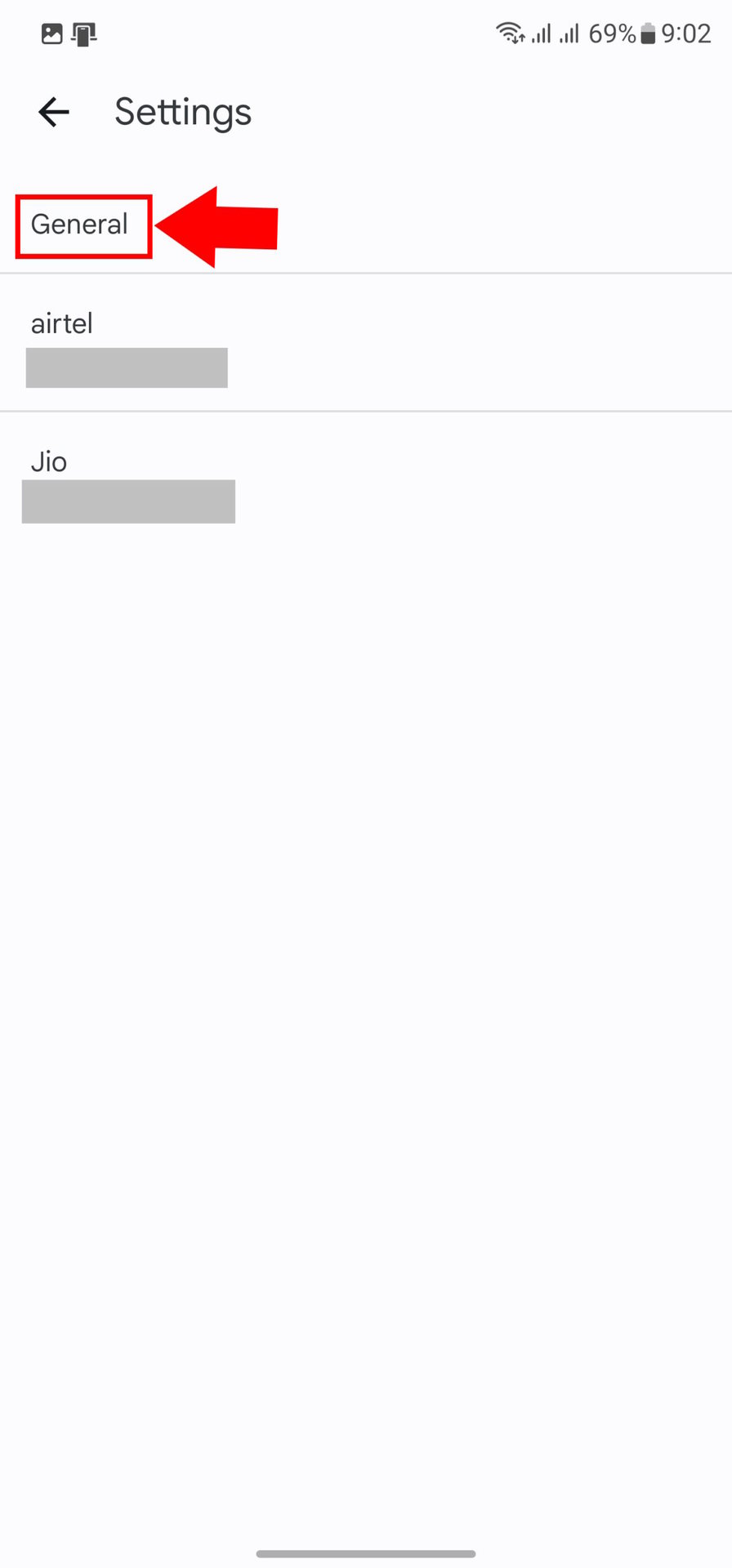This is a detailed screenshot from a cell phone display. At the top right corner of the screen, there are icons showing Wi-Fi coverage, a 69% battery level, and the current time, 9:02. Below this, a black arrow pointing to the left is visible, accompanied by the word "Settings" on the right side of the arrow.

The main section of the screenshot displays a heading labeled "General," which is prominently outlined in a red border with a red arrow pointing towards it. Beneath the "General" heading, the cell phone network service providers "Airtel" and "Jio" are listed, with both names left-aligned. Portions of the screen under these entries are grayed out to preserve privacy.

The background of the image is white, and at the very bottom, there is a short gray horizontal line. The image does not contain any photographic elements, people, animals, birds, plants, buildings, mountains, or automobiles. It is a plain screenshot focusing purely on the phone's settings interface.